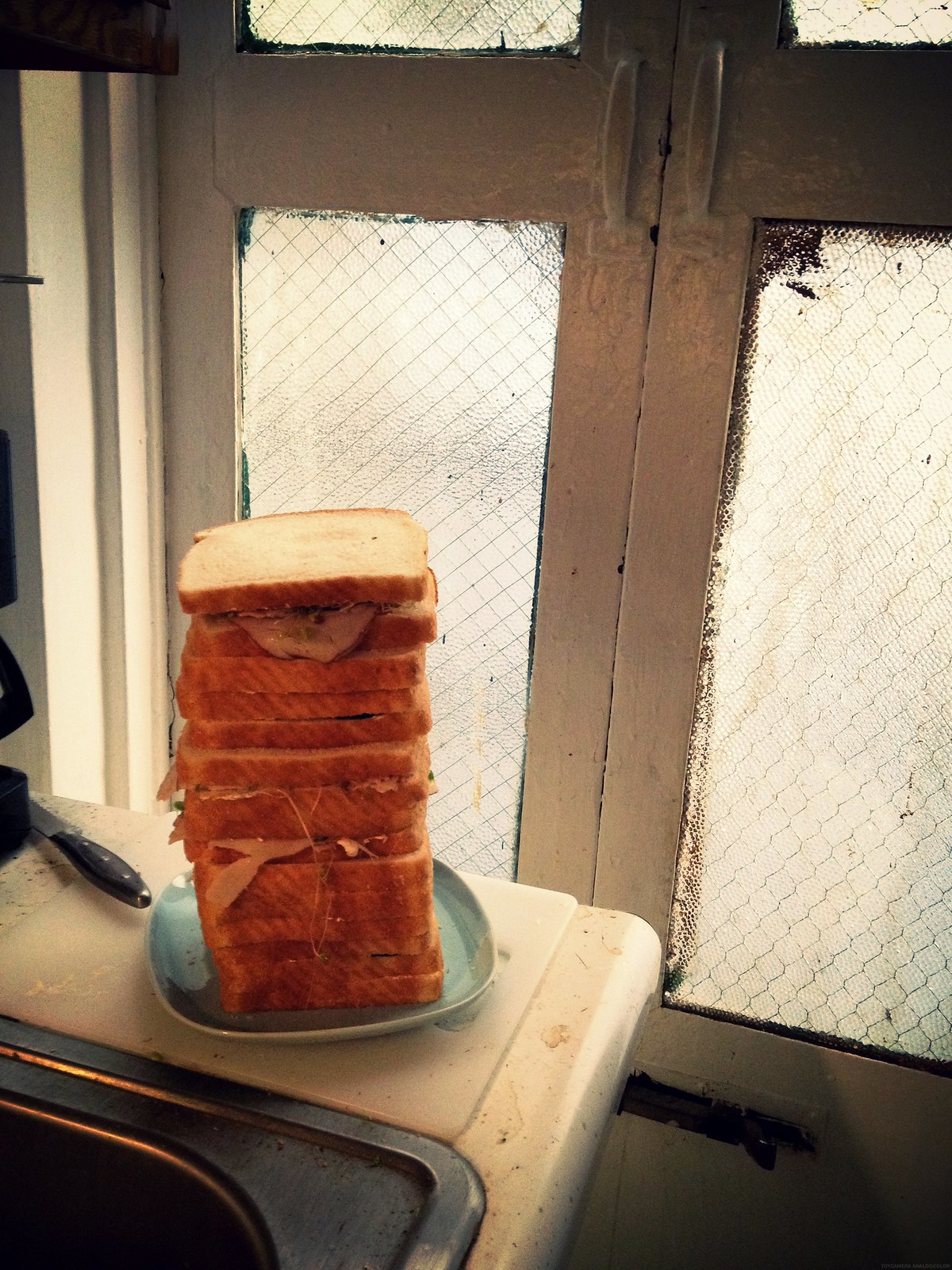The image captures a strikingly tall stack of approximately 20 slices of white bread, each with different fillings and ingredients peeking out from the sides. This towering sandwich creation sits on a rounded square teal plate, which is placed on a white cutting board. The setting appears to be a messy kitchen area, with a dirty, stainless steel sink nearby. The countertop is cluttered and grime-ridden, contributing to an overall sense of disarray. Adjacent to the plate is a knife, hinting at recent sandwich preparation. The background features a large, white-framed window with four panes of glass reinforced with wire mesh, through which muted daylight filters in. Despite the daytime lighting, the image is somewhat dim and shadowy, further highlighting the untidy environment.